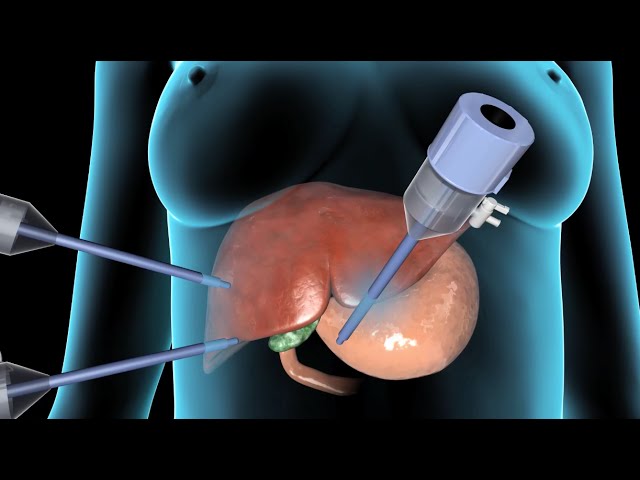The image is a detailed, simulated computer depiction of a medical procedure focused on a woman's abdomen. The background is entirely black, contrasting with the woman's body, which is rendered in a cyan-colored gradient, illuminated to appear almost neon green. The simulation prominently features the woman's torso from below the breasts down to the lower abdomen, with her arms lying at her sides. Within the abdomen, one can identify organs such as the liver, gallbladder, and spleen.

Three conic, needle-like probes are positioned to puncture the body at different points, with two coming from the left side of the image and a third from the center right. These probes are depicted as light blue and seem to be controlled externally, possibly suggesting a scenario for minimally invasive surgery. This high-tech simulation provides a vivid and almost 3D-like x-ray view, emphasizing the precision of the medical instruments and the intricate details of the internal organs.